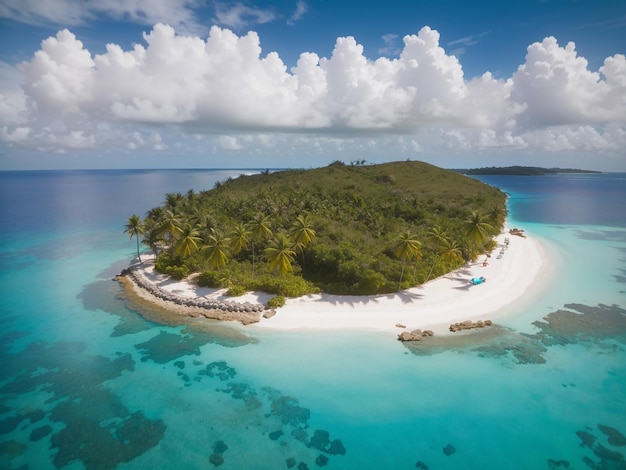This image depicts a small tropical island surrounded by the ocean. The island features dense vegetation at its center, making it virtually impenetrable, with an array of palm trees dotting its periphery. Bright white sand encircles the island, contrasting beautifully with the crystal-clear, turquoise green water near the shore. As the water stretches further into the ocean, it transitions into a deep dark blue, with visible rocks submerged in the shallower areas, showing all the way to the ocean floor. Along one side of the beach, a row of rocks is noticeable, and on the other side, there's a blue object that resembles either a table or a boat. On the sandy beach sits a lone chair, adding a touch of human presence to the natural scene. The sky above is filled with fluffy white clouds with patches of blue breaking through. In the distant background, there's another highly vegetated island, appearing about half a mile to a mile away. The entire scene gives an impression of isolation and tranquility, with no people in sight.